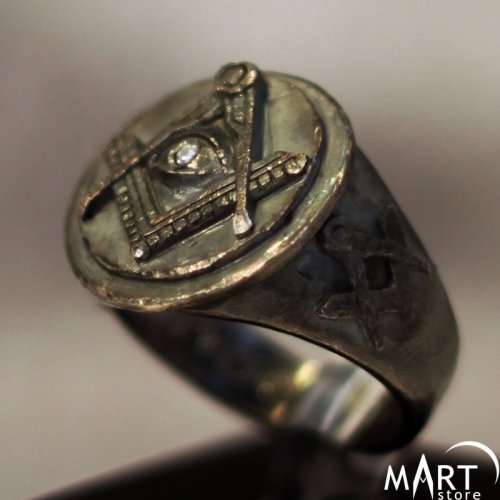This close-up advertisement for Mart Store prominently features a weathered, metallic ring adorned with Masonic symbols. The focal point of the ring's face showcases the iconic compass and square insignia, framing a jewel-encrusted eye. The intricate design reveals triangular shapes pointing in opposite directions, embodying the distinctive Masonic aesthetic. With its rough, tarnished surface, the ring exhibits a unique greenish-gray patina, accentuated by worn silvery areas, enhancing its antique allure. The setting is brightly lit, contrasting the detailed ring against a brown and white backdrop with a grayish hue. The bottom right corner of the image prominently displays the Mart Store logo and name in white, accompanied by a crescent moon symbol. The overall clarity of the image emphasizes the intricate craftsmanship of the ring and its vintage appeal.